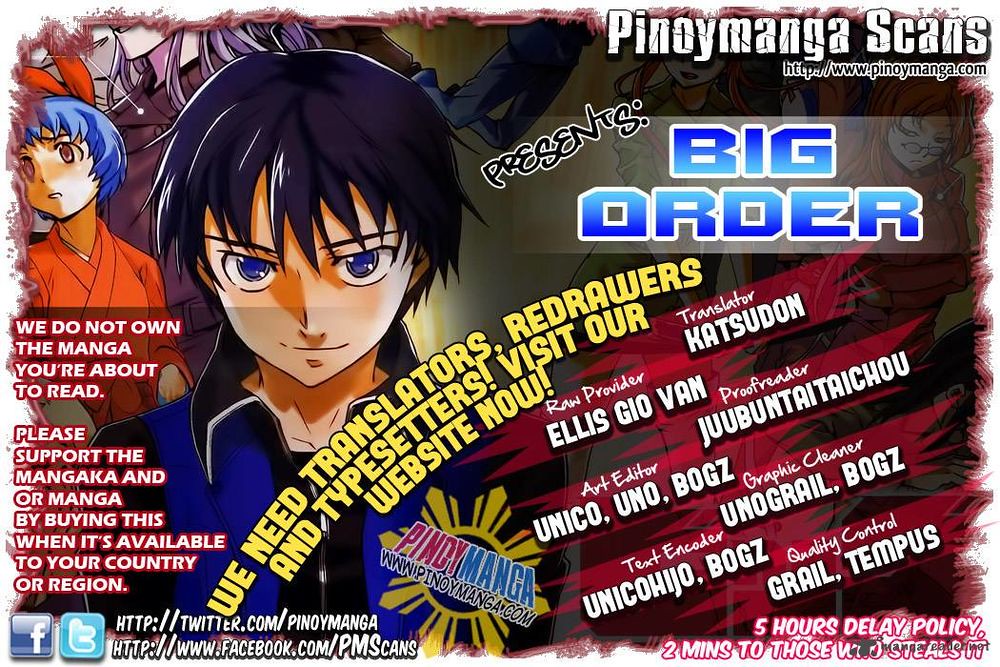The image appears to be a digital advertisement for an anime, specifically promoting a manga titled "Big Order" by Pinoy Manga Scans. The background features two anime characters: one wearing a red jacket with blue hair and another larger figure adjacent to it with blue eyes and black hair, adorned in a black and blue jacket. At the top right corner, it is labeled "Pinoy Manga Scans" with the website URL www.pinoymanga.com beneath it. 

Prominently displayed in the center with yellow lettering, the ad states, "We need translators, redrawers, and typesetters. Visit our website now," alongside a comprehensive list of contributors: Translator (Katsudon), Raw Provider (Alice Giovann), Proofreader (Ubuntatai Kato), Art Editors (Unico, You know, and Box), Graphic Designer (Unigrill, Box), Test Encoder (Unico, Hejo, Box), and Quality Control (Grey and Tempest). 

A cautionary message reads, "We do not own the manga you're about to read. Please support the mangaka and/or manga by buying this when it's available in your country or region," underscored by Facebook and Twitter logos directing to twitter.com/pinoymanga and facebook.com/PMSscans. The ad concludes with a “five-hour delay policy” statement at the bottom right corner, emphasizing "two minutes to those who steal it."